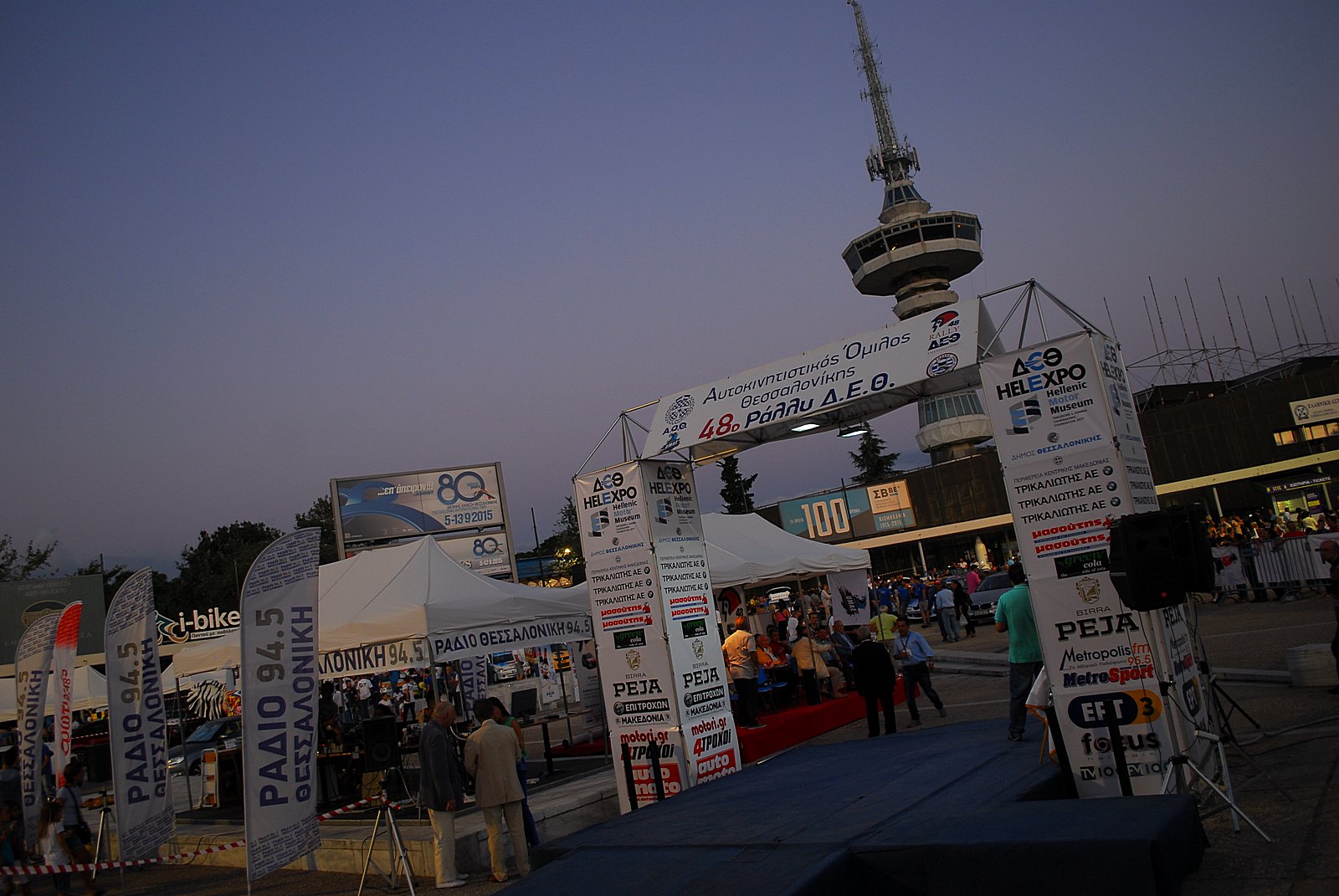The photograph depicts a lively fair or expo taking place in the evening, with the sky transitioning into dusk. The scene is bustling with people walking around numerous white tents. A significant landmark in the background resembles the famous London Post Office Tower, though its presence casts doubt on the exact location due to the Greek and possibly other foreign text on the signs. Prominent signage includes terms like "H-E-L-E-X-P-O," "Hellenic Motor Museum," "Pija," "Metropolis Metro Sport," and "I-Bike." The entrance of the fair is adorned with a blue carpet and a paper archway, giving it an inviting appearance. Some attendees are dressed in suits, adding a touch of formality to the otherwise festive atmosphere.